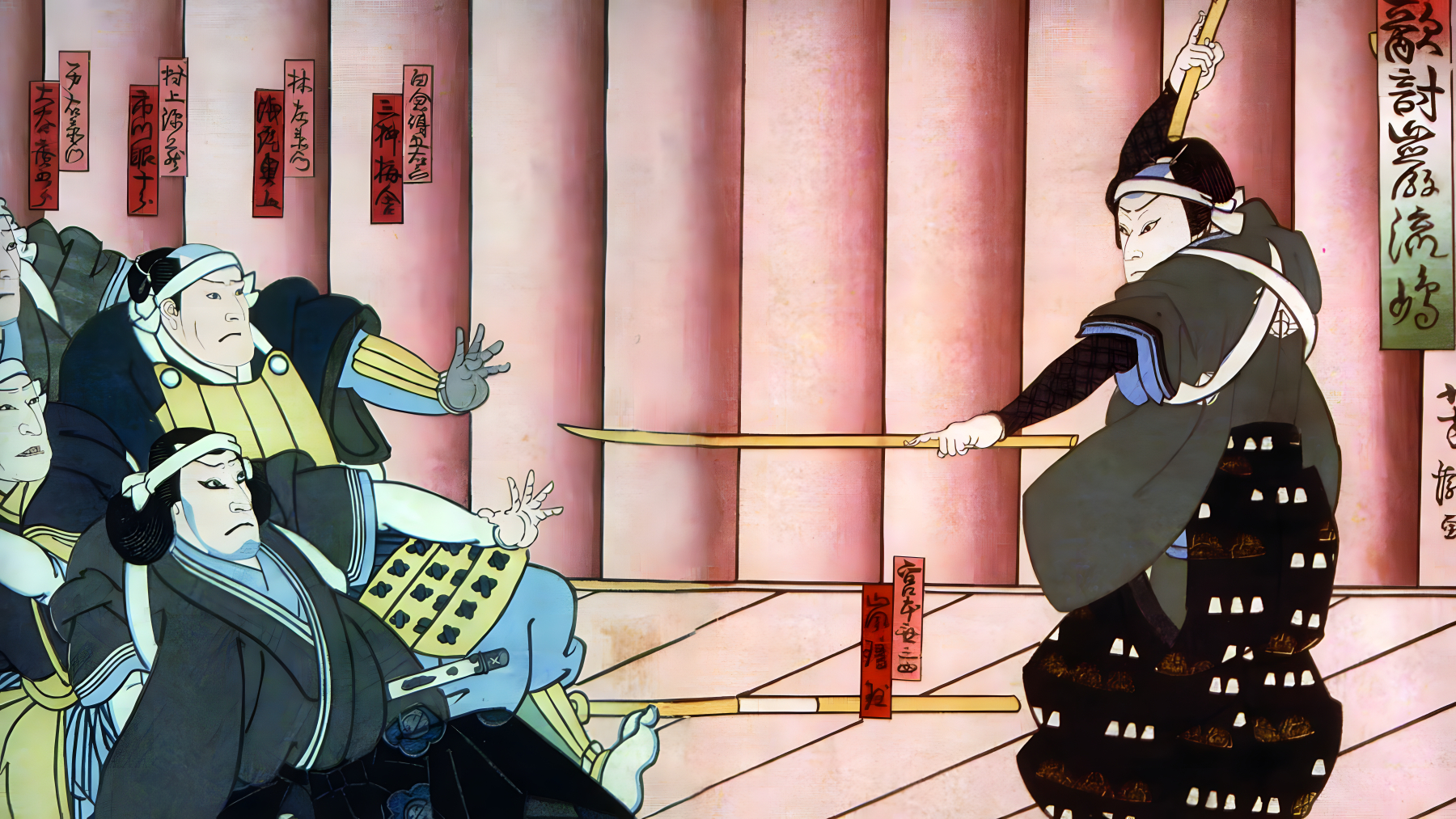The image appears to be an intricately detailed scene from an Asian animated comic strip, likely of Japanese or Chinese origin, featuring vibrant colors typically found in anime or oriental cartoon drawings. The scene is set against a pink background with walls and pillars, some of which have darker pink shading, and the floor is depicted with wooden planking.

At the center of the action is a warrior standing on the right, distinguished by a gray cloak, a black skirt, and black hair. He wields what appear to be yellow-colored sticks or swords and is in a dynamic pose, raising a spike towards other figures. The warrior seems to be the focal point, causing the other three or four men, dressed in traditional Asian attire, to lean back with expressions of fear as they have fallen or are crouching on the floor. A yellow stick is also seen fallen on the ground.

The background is adorned with multiple banners featuring Japanese or Chinese writing in various shades of pink and red. These banners hang predominantly on the far right and left sides of the image, adding to the rich cultural ambiance. The overall style of the artwork suggests it could be reminiscent of old print artwork, possibly watercolor, embodying a historical or traditional aesthetic.